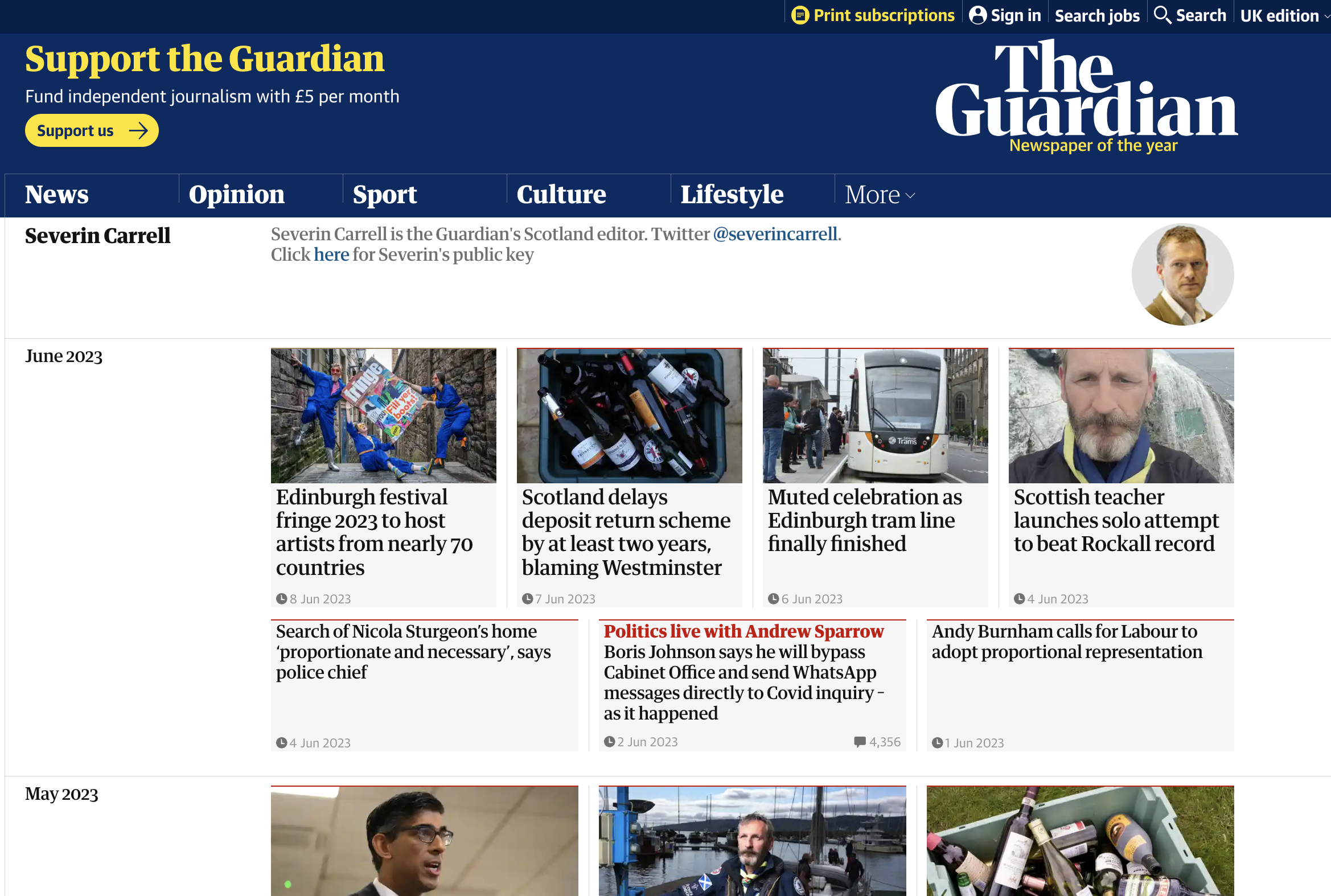This screen capture showcases the homepage of The Guardian's website, viewed on either a computer or tablet. The top right corner features user-centric options such as print subscriptions, sign-in, job search, general search, and an indication that it is the UK edition of The Guardian. 

To the left, on the top blue ticker bar, there's a button inviting users to support The Guardian. The right side of the same bar prominently displays "The Guardian - Newspaper of the Year." Below this, the navigation menu offers categories such as News, Opinion, Sports, Culture, Lifestyle, and a "More" option for additional sections.

Further down, the homepage organizes headlines chronologically. The section for June 2023 features seven headlines, four of which are accompanied by relevant images. Following this, the May 2023 section includes various headlines displayed with three associated images, providing a visually engaging overview of past news.